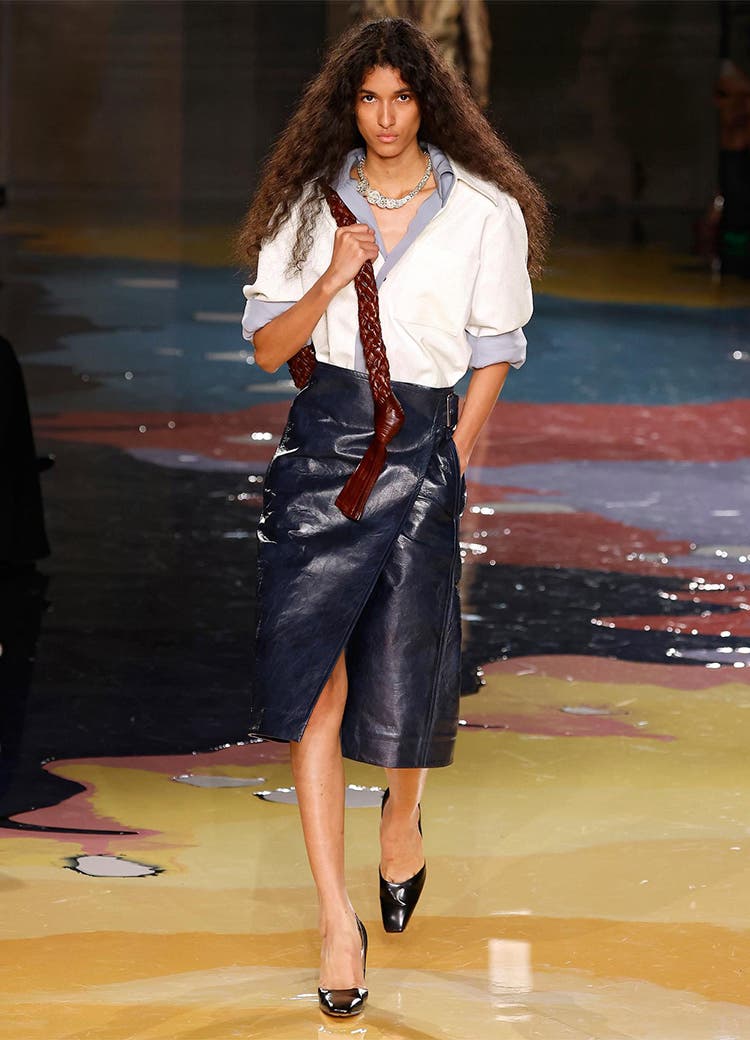In this photograph, a tall and slender model with long, wavy, and voluminous light brown hair walks down a unique and vibrant runway. The runway itself is notably distinctive, featuring a multicolored floor with a predominant yellow base accented by splatters of dark purple, pink, blue, and light purple. The model exudes a serious demeanor as she struts confidently. She is adorned in a contemporary ensemble that includes a white blouse with a blue collar and blue cuffed sleeves. Around her neck, she sports a chunky, bright necklace which adds a touch of boldness to her look. 

Her lower half is dressed in a dark blue leather wrap skirt with a modest slit that extends past her knees, showcasing her bare legs. She carries a brown leather-strap bag slung over her shoulder, though the specifics of the bag remain partially obscured. On her feet are black high-heeled shoes, which appear slightly ill-fitting as her toes are visible peeking out from one of them. This stylish yet somewhat imperfect appearance adds a touch of realness to the high-fashion scene captured in this runway image.